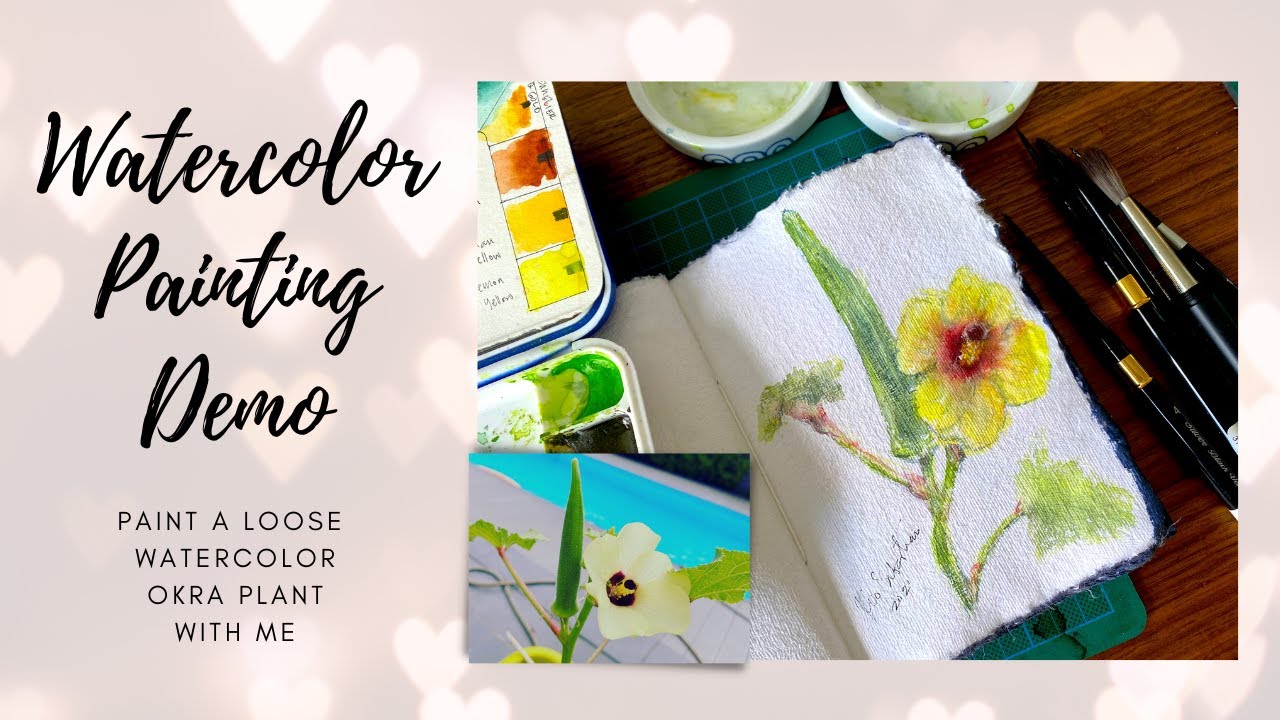This advertisement features a detailed demo for a watercolor painting, highlighted on a grayish-tan background adorned with white hearts. The primary text, "watercolor painting demo," is written in cursive in black, followed by the printed phrase, "paint a loose watercolor okra plant with me." On the right side, a guidebook for paint palettes and a paint box lid with various color samples are depicted, set against a brown table. Inset within this image is a color photograph of an okra plant featuring white flowers, green stems, and a blue background, possibly a pool. 

To the left, the main image showcases a watercolor painting of an okra plant on soft, white felt paper. The plant has five yellow petals with a purple center and green stalks with leafy extensions. Additional elements include paintbrushes, a green mat partly obstructed by the painting, and a palette containing mixed paints, notably lime and dark green hues. The painting scene is set beside some other books and art supplies, enhancing the creative workspace ambiance.